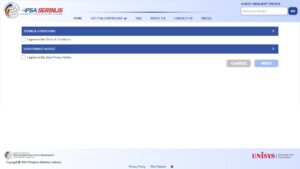The image features a top header with a gradient background transitioning from white on the left to light blue on the right. Positioned towards the left is a light gray globe icon, accompanied by a curved blue area arching above it, followed by a shorter, curved orange section intersected by a black line. On the right side of the header, there is a slightly blurry logo due to image compression, which appears to have the initials "PSA" in blue block letters. To the right of this, the text "SERBILIS" appears in the same font but in red lettering.

Centered at the top, there is a divider line, light gray on the sides and transitioning to a darker gray in the middle, creating a 3D effect. Below this divider, a menu bar spans the width of the image. Each menu option is in dark blue capitalized font, with "HOME" likely listed as the first option on the left and "SEARCH" as the last option on the right.

The main content area below the menu features a large white rectangular section. At the top of this section, a long dark blue rectangular header with white text aligned to the left stretches across. On the far right of this blue header, a white arrowhead points to the right. Beneath this header, there's a white background with a small checkbox to the left and some small black text beside it.

This pattern repeats further down with another elongated dark blue rectangular icon with white text to the left and a white arrowhead to the right. Again, beneath this header, there's a white background with a checkbox to the left and small black text to the right.